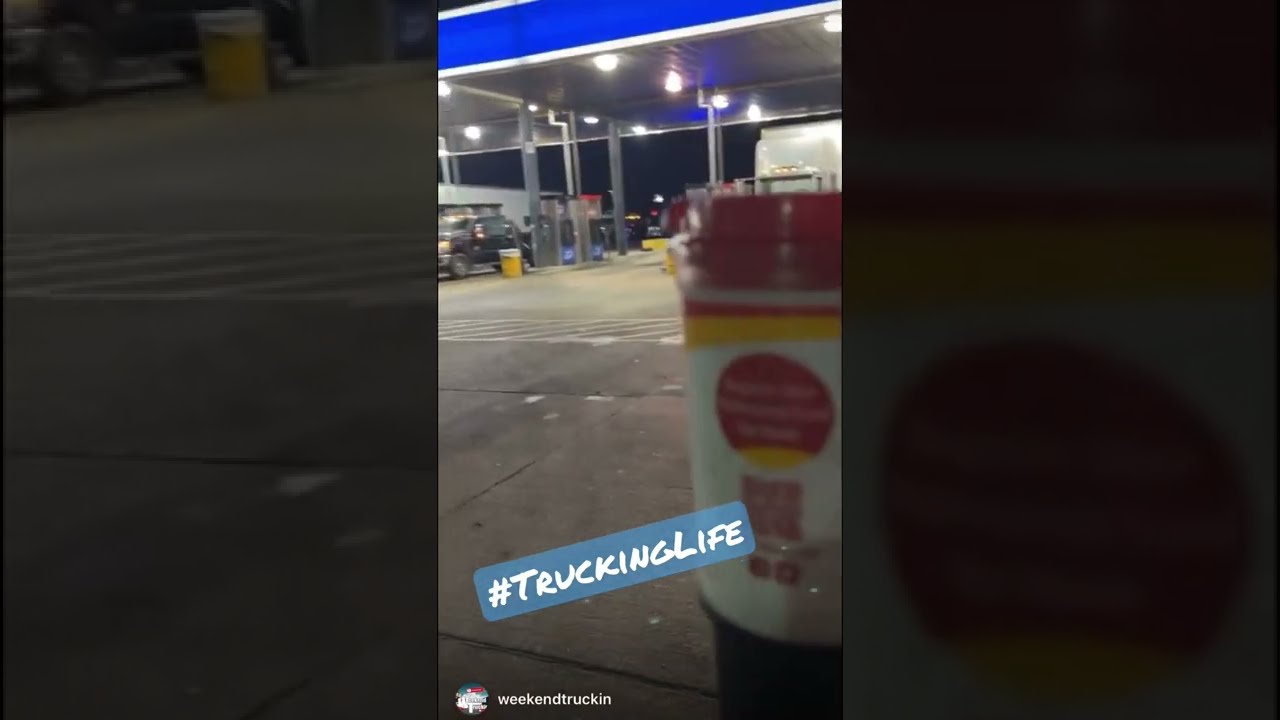The photograph captures a nighttime scene at a gas station, dimly lit under an evening sky. Central to this image is the illuminated gas station awning covering several fuel pumps, with various vehicles, including a couple of 18-wheelers and a passenger truck, positioned around the area. Prominently displayed at the bottom middle of the photograph is a blue rectangle with white text that reads "#truckinglife," alongside the phrase "weekend trucking." A close-up of a coffee cup is positioned nearby, suggesting it’s taken from the perspective of someone inside a vehicle. The entire image is framed by a black border, with blurred, enlarged elements of the central scene on either side, emphasizing the focus on the gas station at the center.